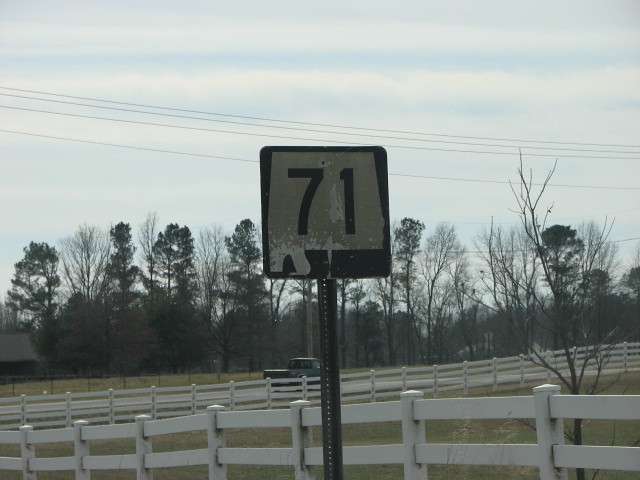In this photograph, the serene backdrop showcases expansive farmland with a mixture of conifer and pine trees dotting the horizon. Nestled in the far-left corner, a quaint barn can be seen in the distance, adding a rustic charm to the scene. Dominating the center is a weathered Route 71 street sign, its white face and black lettering partially obscured by splatters of paint. Behind the sign, a white fence stretches horizontally, extending further back into the background. A turquoise Ford F-150 truck travels eastward along a road that cuts through the lush grasslands. A solitary tree stands just behind the first section of the fence on the bottom right-hand side, contributing to the tranquil rural atmosphere.